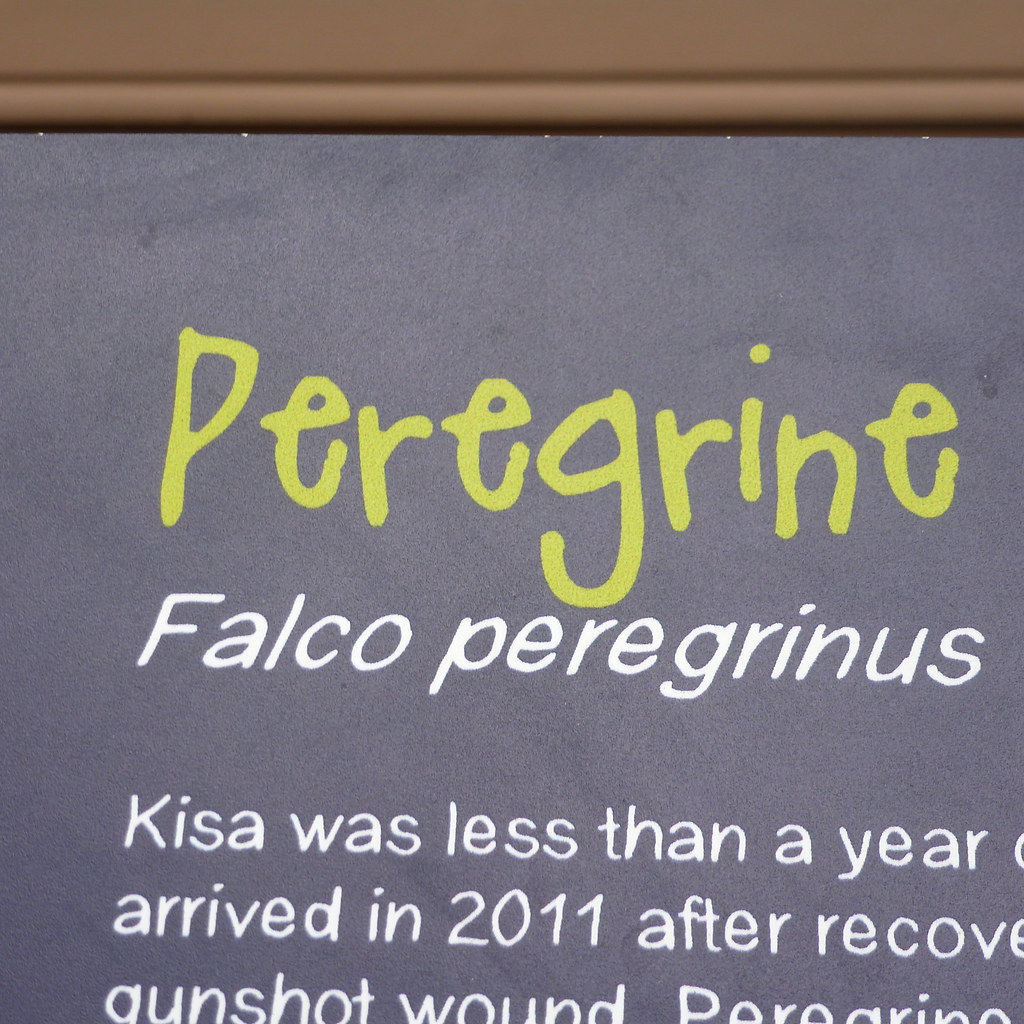The image shows a black background with a partial display of text. At the top, there is a single line of yellowish lettering that reads "Peregrine, P-E-R-E-G-R-I-N-E." Below this, in white letters, it says "Falco Peregrinus, F-A-L-C-O P-E-R-E-G-R-I-N-U-S." Additionally, the remaining visible white text provides limited information: "Kissa, K-I-S-A, was less than a year, arrived in 2011 after recove[r]y, gunshot wound." The text is cut off on the sides and towards the end, leaving incomplete phrases. At the very top, above the main text, there appears to be a textured, brown border reminiscent of a floor sideboard.